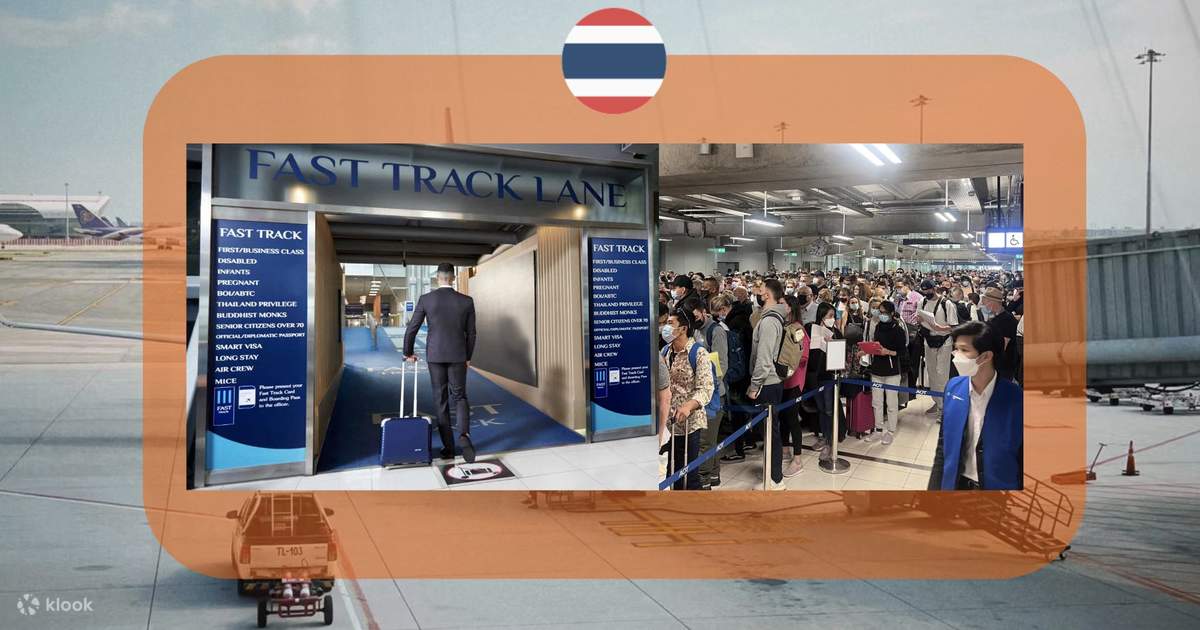The photograph features a two-image collage set against the backdrop of an airport runway, complete with a truck towing cargo and planes in the distance. Dominating the center of the composition is an orange-bordered section with the Thai flag symbol atop. The left image captures a serene, empty hallway labeled as the 'fast track lane' where a lone man, possibly a pilot clad in a black suit and pants, strides effortlessly, pulling his blue rolling luggage. The corridor is flanked by blue signs with the 'fast track' label prominently displayed. In stark contrast, the right image portrays a chaotic scene of dense crowds lined up in numerous rows at the security gate, filled with people wearing masks, and carrying backpacks and luggage. The watermark "KLOOK" can be seen in the bottom left-hand corner.